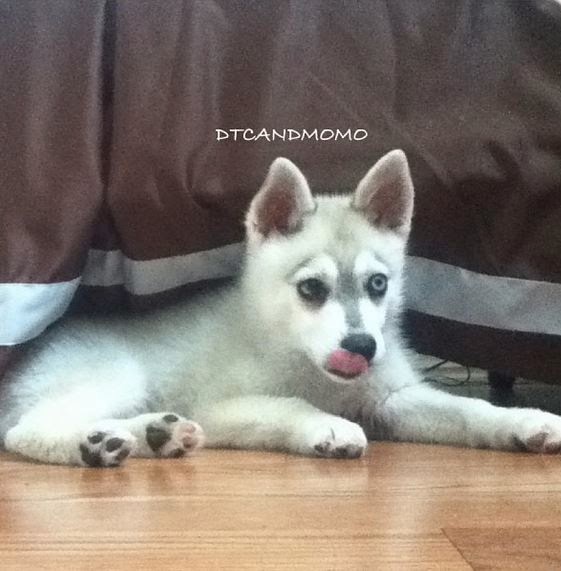This captivating photograph showcases a delightful young husky puppy, estimated to be around three months old, lying down on a brown hardwood floor beneath a brown tablecloth with a thick white stripe running along its bottom edge. The puppy's coat is primarily white, with gray accents on its nose, the top of its head, and a faint gray along its back. Its expressive eyes are a pale gray with striking black irises, adding depth to its innocent gaze. The puppy's ears are upright, revealing a hint of pink within. Its black nose is playfully being licked by a pink tongue, capturing a moment of pure, endearing behavior. The four paws are particularly detailed; the front ones are entirely white, while the back paws display black and pink pads, adding to the puppy's unique charm. This serene scene is anchored by the cozy, brown tablecloth draped above, providing a warm, inviting atmosphere as the puppy lounges comfortably.